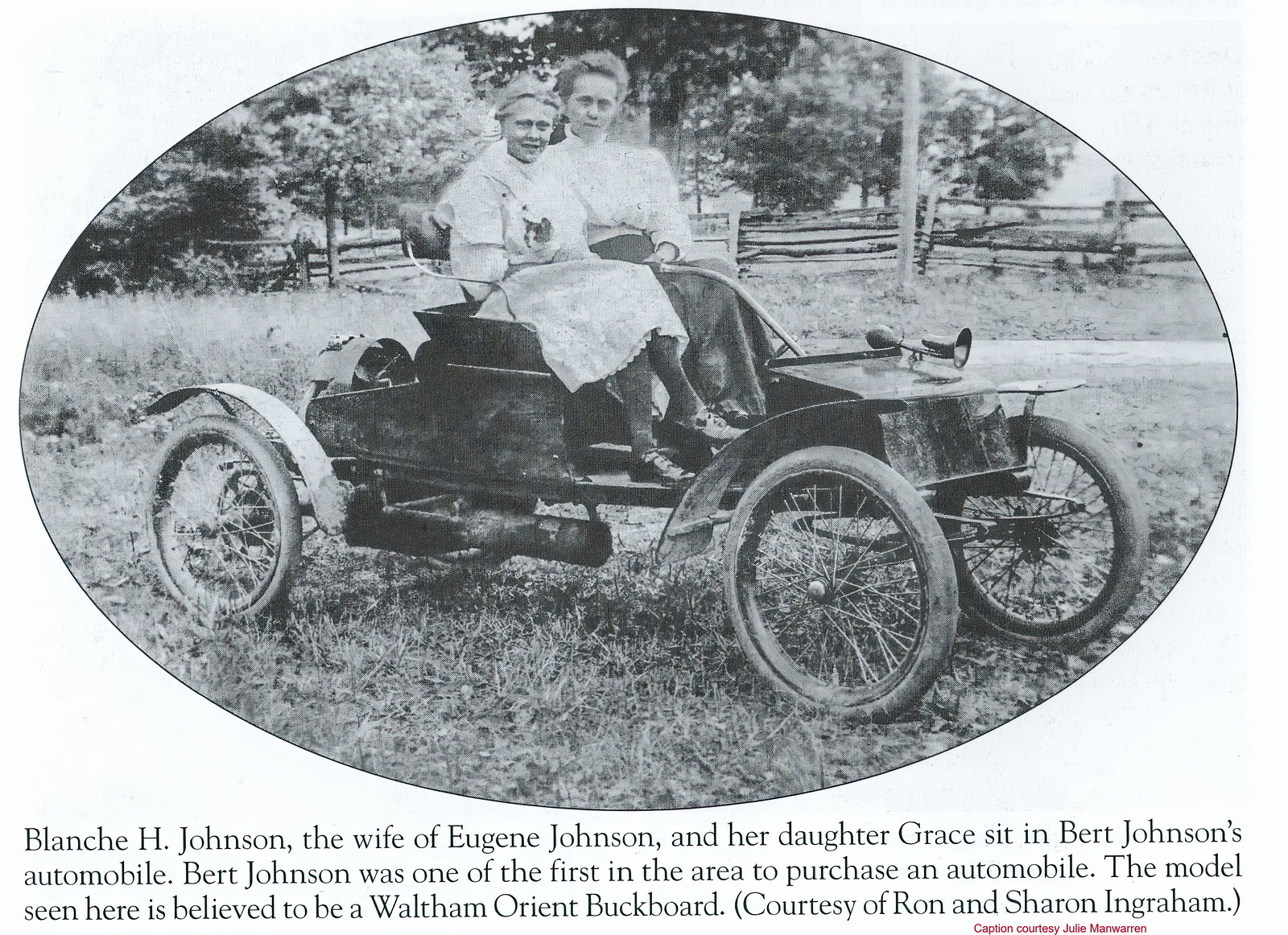A beautifully vintage, black-and-white photograph, likely from the 1920s, captures two young women sitting in an open-air automobile, possibly a Waltham Orient Buckboard, with the car's top removed. The image is enclosed in a horizontally aligned oval frame. The young woman on the left, who appears to be blonde and is smiling, sports a rolled and swept back hairstyle characteristic of the 1920s. Both women are dressed in white, with the one on the left in a slightly shorter light-colored dress paired with dark shoes and stockings, and the one on the right in a long dark skirt and white top. The car, positioned on a grassy area, features wheels reminiscent of modern fat-tire bike wheels. A distinct, old-fashioned horn is visible at the front of the car. The background depicts a picturesque scene with trees occupying the top third of the image, a wooden fence with three horizontal slats, and higher grass up to the left behind the vehicle. A path can be seen behind the car to the right. Beneath the oval image, in Times New Roman font, is the caption: "Blanche H. Johnson, the wife of Eugene Johnson, and her daughter Grace sit in Burt Johnson's automobile. Burt Johnson was one of the first in the area to purchase an automobile. The model seen here is believed to be a Waltham Orient buckboard, courtesy of Ron and Sharon Ingraham." Additionally, in small red writing printed in Comic Sans, there is a secondary credit: "captions courtesy of Judy Ingram."